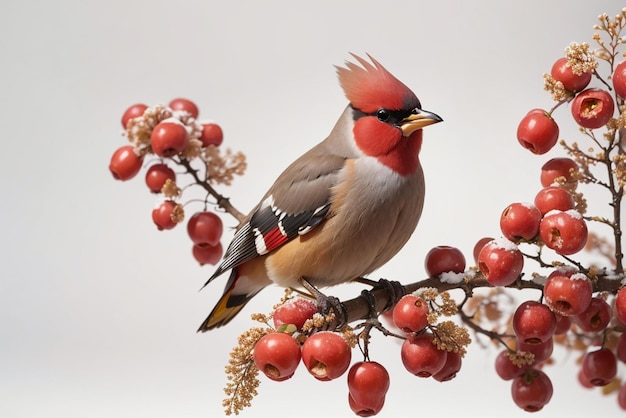This image is a highly detailed, realistic depiction, possibly created using computer-generated techniques, hand-drawing, or painting, with a smooth, animation-like style. The background is off-white, lending a serene and calm atmosphere to the scene. The focus of the picture is on the right where a snowy branch, resembling a holly branch, holds clusters of small red berries and a small brownish-orange piece of foliage.

Perched on the branch is a bird that closely resembles a cardinal, specifically a female cardinal, featuring prominent and intricate feather details. The bird showcases a white chest and light tan stomach, with a back covered in light brown feathers. Its wings display a beautiful pattern of black, red, and white feathers, while its head is strikingly red adorned with a black stripe across the eye area. The bird's beak is yellow with a distinct black streak running from the top of its head to the tip of its beak. The cardinal is oriented towards the right, integrating harmoniously with the vibrant yet delicate tones of the berries and the snowy ambiance of the branch.